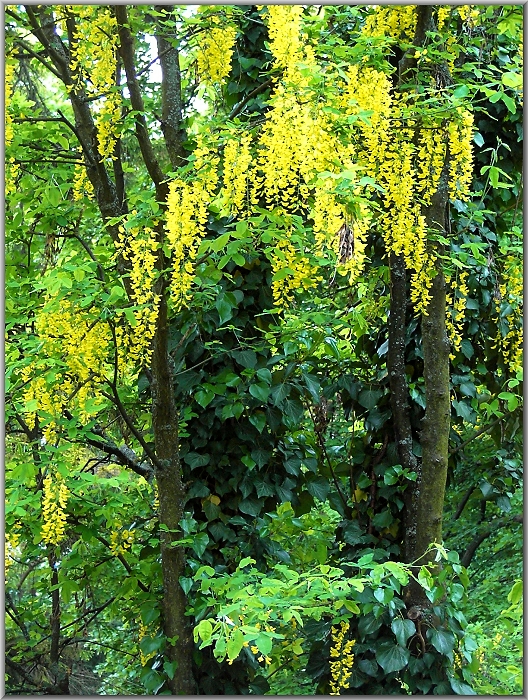The image captures an enchanting outdoor woodland scene bathed in the vibrant colors of spring. The focal point is two slender, youthful trees at the center, each standing six to eight feet tall, with trunks about the diameter of a baseball or softball. Surrounding these trees is an abundance of lush, green vegetation interspersed with clusters of vivid, long, dangly yellow flowers. These striking flowers, seemingly sprouting from a series of vines entwined around the trees, hang gracefully, creating a cascade of color from the tree tops. The scene exudes a fresh, slightly damp atmosphere typical of spring, with the green and yellow hues dominating the composition, embodying a pure, vibrant burst of nature.